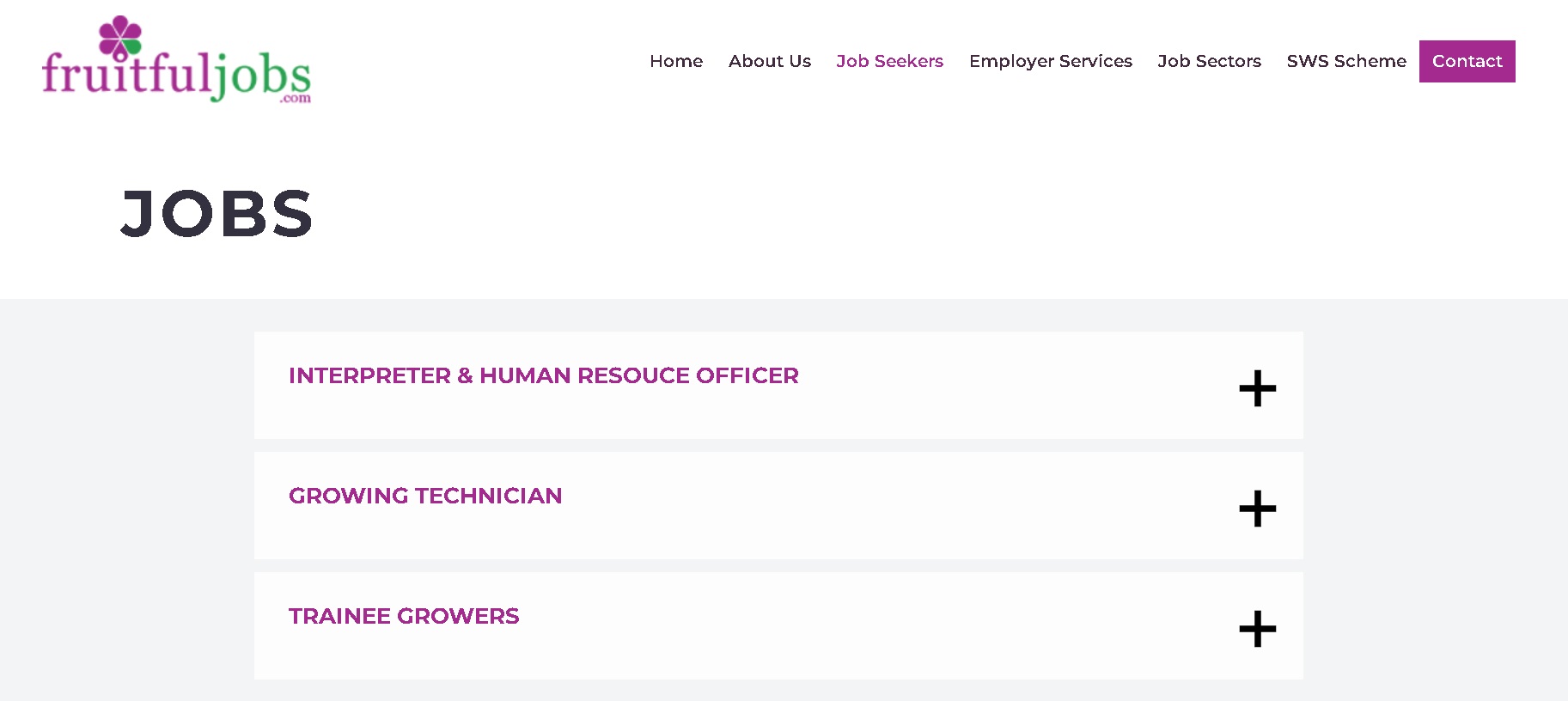The image from the website labeled "Fruitful Jobs" features a vibrant and informative layout. At the top of the image, the word "Fruitful" is prominently displayed in bold purple letters, accompanied by a colorful flower where each petal is purple except for one green petal. Below this, the word "Jobs" is written in a striking green font, and underneath, "JOBS" is emphasized further in large black letters.

Across the top navigation bar, a series of clickable options are presented, including "Home," "About Us," "Job Seekers," "Employer Services," "Job Sectors," "SWS Scheme," and "Contract." The "Contract" section is highlighted in a purple box with white text.

Further down the page, there is a gray box featuring job titles in purple text, each accompanied by a plus sign for additional details. The job titles listed include "Interpreter and Human Resource Officer," "Growing Technician," and "Trainee Growers." Once the list of job titles ends, there are no further descriptions available within the visible portion of the box.

Despite the detailed layout and clear categorization of job titles, the image does not provide a specific description of what services or roles "Fruitful Jobs" offers, leaving the viewer to seek more information to understand the site's purpose fully.